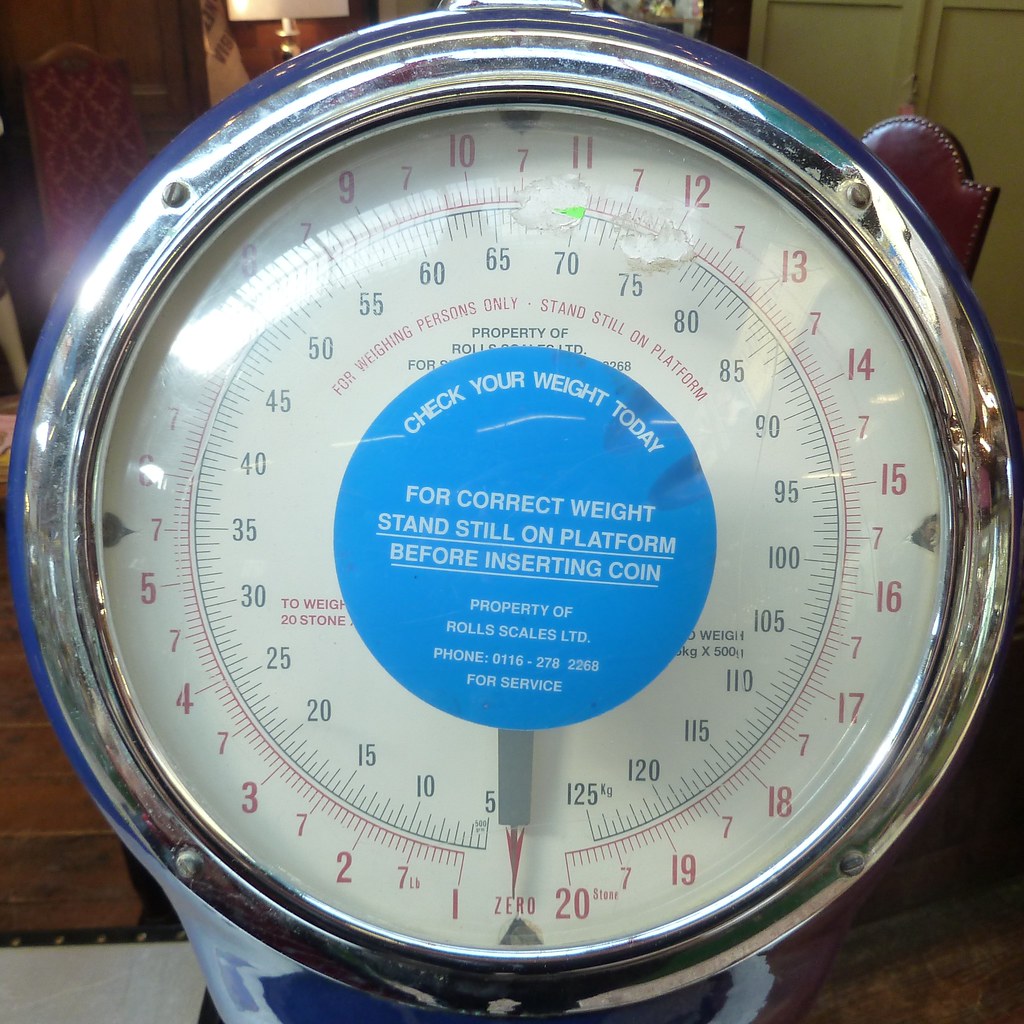This photograph features a vintage, circular weighing meter prominently displaying intricate detailing. The scale's boundary is metallic and silver in color, encasing a transparent glass through which the measurement numbers are visible. There are dual sets of numbers: red digits ranging from 1 to 20 pounds on the outer circle, and black digits indicating weights from 5 to 125 kilograms on the inner scale. The meter is currently set to zero.

Centrally positioned on the glass is a blue, circular sticker with white text that reads: "Check your weight today. For correct weight, stand still on the platform before inserting coin. Property of Rolls Scales Limited, phone 0116 278 2268 for service." This points to its use in public spaces, where users can insert a coin to get their weight measurement.

The background suggests an indoor setting, with visible elements like older leather chairs, a lamp, wooden paneling, and a wood floor, hinting at a possible antique store, leather shop, or restaurant. The scales' blue metal finish with chrome trim and screws, combined with the functional and decorative elements, adds to its vintage charm and precise craftsmanship.